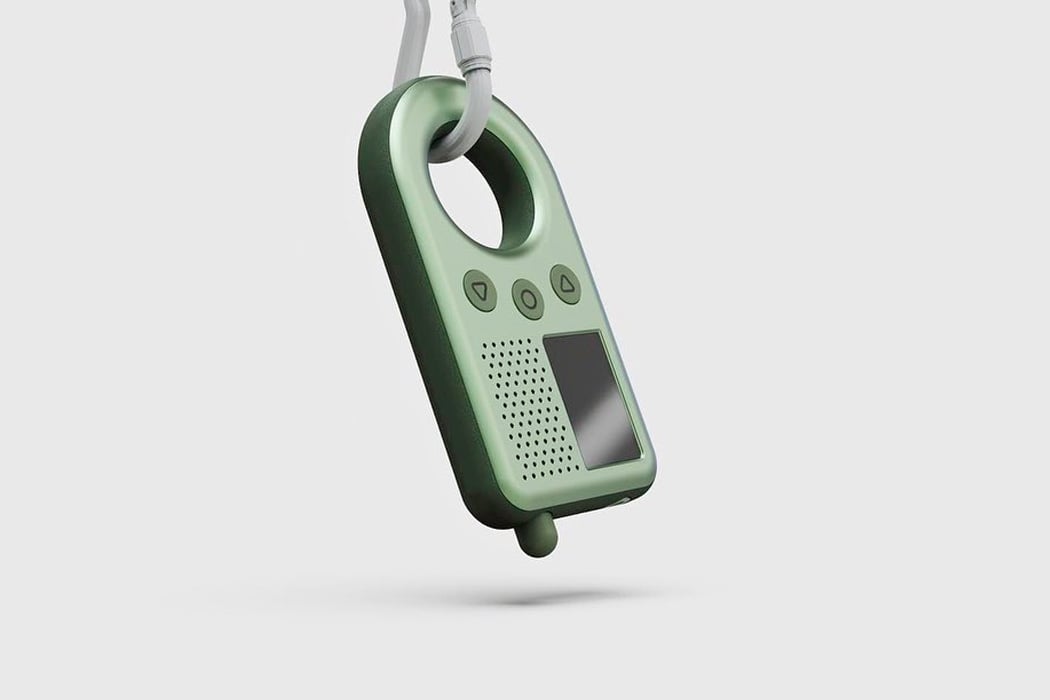This detailed digital rendering visualizes a compact green electronic device, potentially a speaker, music player, phone, or alarm, intricately designed with metal elements. The device features a black screen situated closely to small speaker holes on its lower left side. On its surface, three buttons in a darker green form a half-circle configuration: a downward-pointing triangle, a circle, and an upward-pointing triangle. This dome-shaped gadget, highlighted by its light to darker green color gradient on the edges, is suspended from a white hook via a small hole at its top. The hook does not form a complete circle and secures the device through the small hole at the top, presenting the device as if it is hanging or dangling. The device also seems to have a small antenna and is clipped to a white metal clip. The background setting is minimalist, featuring a gray-white color which ensures focus remains entirely on the suspended device.